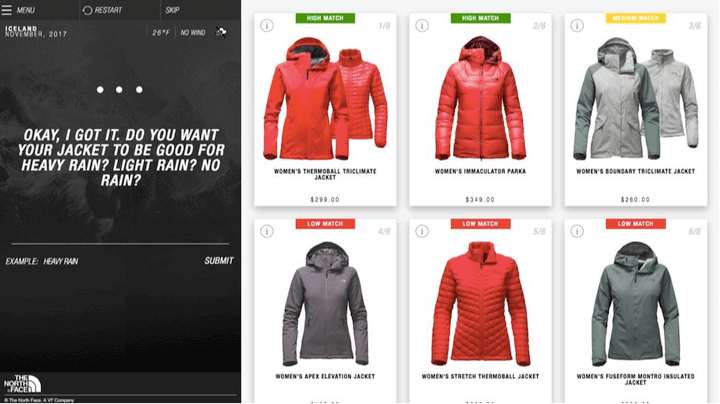The image presents a selection of outerwear and sweaters, categorized in terms of their suitability for various weather conditions. On display are jackets and sweaters in shades of red, blue, and gray. There are multiple red jackets and gray jackets, designed for different intensities of rain—from heavy to light—as well as for dry conditions. Sweaters are also showcased in red and gray hues, providing options for layering in cooler, dry weather. The arrangement emphasizes the variety in design and color, catering to diverse style preferences and weather preparedness.